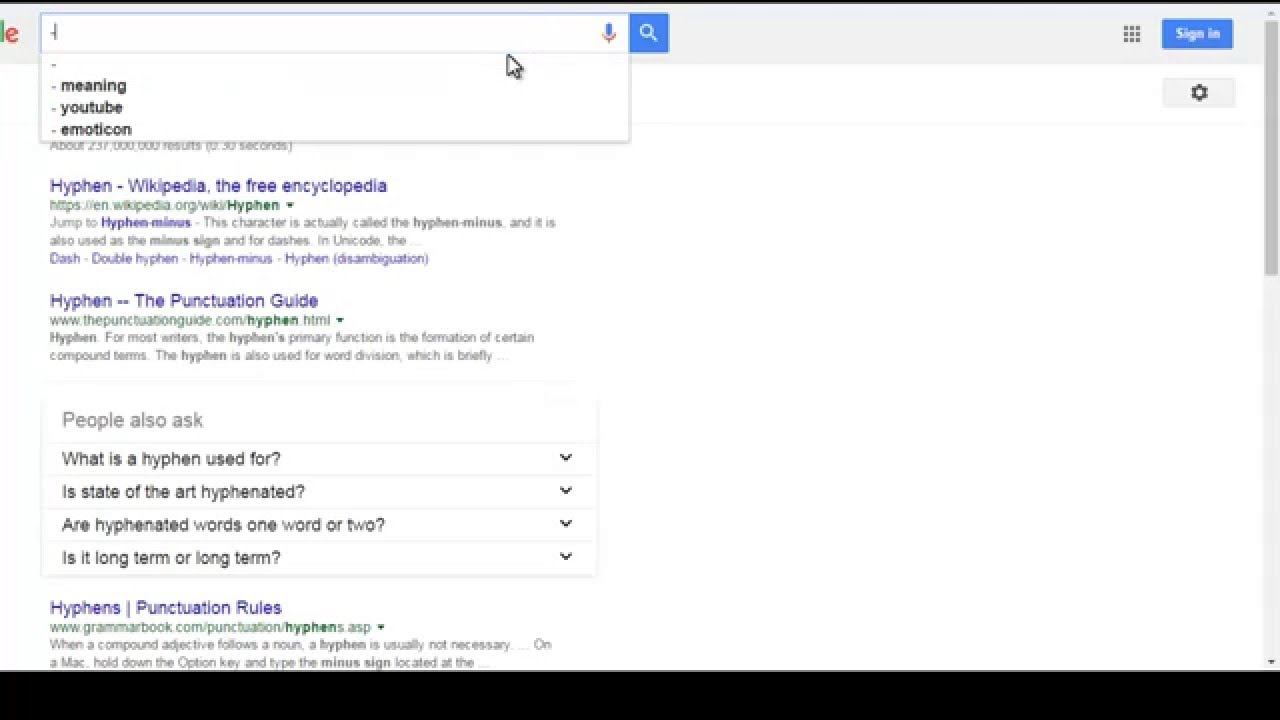The image depicts a Google search results page with a focus on the search bar at the top, where a single character, a hyphen or dash ("-"), has been entered. The resultant suggested searches beneath the search bar include "hyphen," "hyphen meaning," "hyphen YouTube," and "hyphen emoticon." The search results themselves show the top two hits: the first being a link to the Wikipedia page on hyphens, titled "Hyphen - Wikipedia, the free encyclopedia," and the second link leads to "The Punctuation Guide" concerning hyphens. 

Below these primary results, there's a "People also ask" section with FAQs featuring: "What is hyphen used for?", "Is state-of-the-art hyphenated?", "Are hyphenated words one word or two?", and "Is it long-term or long term?" Additionally, towards the bottom of the page, there is another link titled "Hyphens - Punctuation Rules." 

The overall context suggests someone was searching for information about the usage and rules pertaining to hyphens.